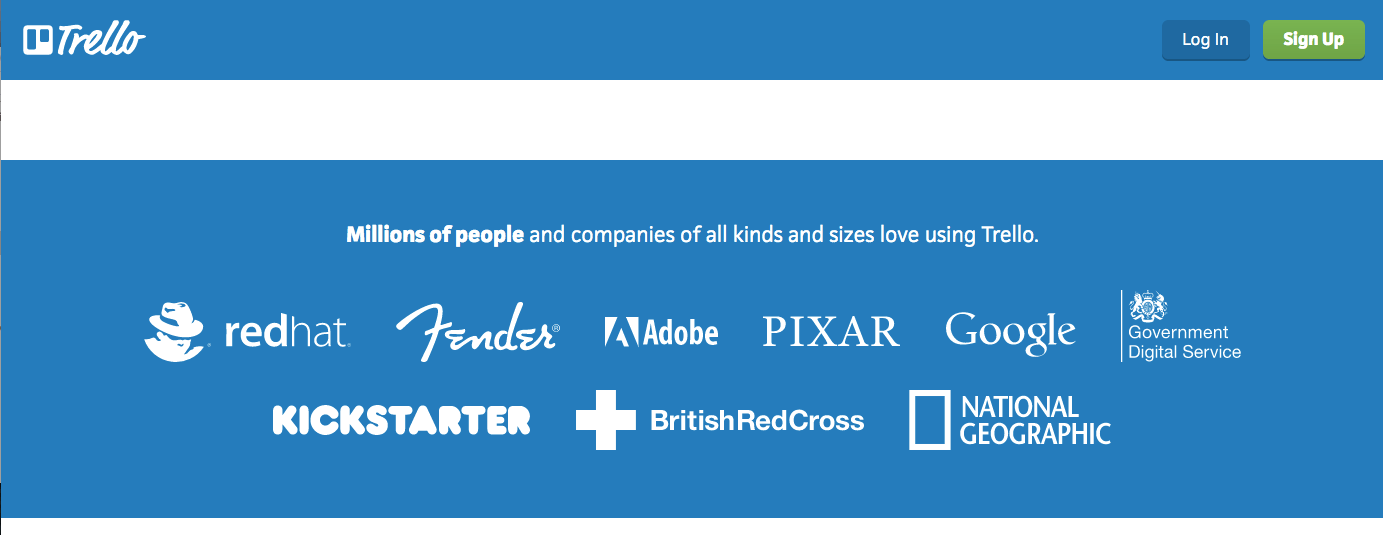This image is a horizontal rectangle divided into multiple sections. The top portion of the image features a vibrant turquoise-blue banner, stretching from left to right. In the upper left corner of this banner, the word "Trello" is prominently displayed in white font, beginning with a capital "T" followed by lowercase "rello." To the left of the word "Trello" is the company's recognizable logo.

On the far right side of the blue banner, there are two buttons. The "Login" button is navy blue with white text, while the "Sign Up" button is green with white text.

Beneath the blue banner, there is a white section of equal size, stretching horizontally across the image.

The largest section of the image, positioned beneath the white strip, features a background graphic with a central focus on text. In bold white font, the headline reads, "Millions of people." Directly beneath this headline, in a non-bolded white font, the text continues, "and companies of all kinds and sizes love using Trello."

Below this text, a series of company logos are displayed, arranged in two rows. The first logo features an image of a person wearing a hat, likely representing a specific brand or company. Following this, the logos for well-known companies such as Red Hat, Fender, Adobe, Pixar, Google, and Government Digital Service are shown. The second row includes logos for Kickstarter, British Red Cross, and National Geographic. This arrangement underscores Trello's widespread usage and popularity among diverse organizations.